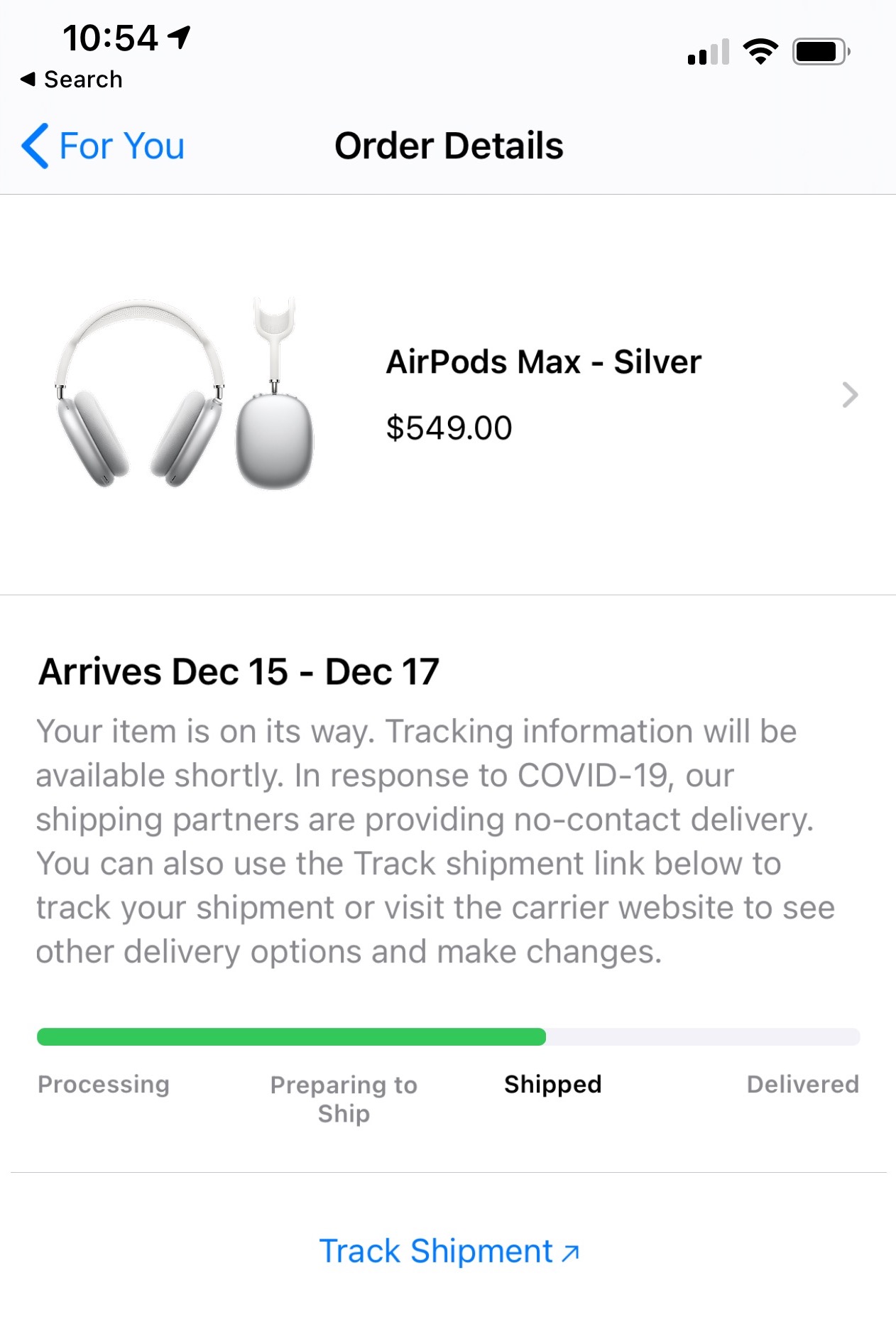The image depicts an online purchase confirmation screen with various status indicators displayed on a white background. 

In the upper left corner, the time is shown in black as "10:54," accompanied by a location arrow icon. Further to the right, the cellular signal bars are depicted with two black bars and two gray bars. Next to this, the Wi-Fi icon displays three fully illuminated bars, and just to the right of that is the battery icon, which is mostly black, indicating partial battery life.

On the left side of the screen, below the status icons, there is a left-facing arrow labeled "Search." Directly beneath this arrow is another left-facing arrow in blue labeled "For You." Centered on the screen, the text "Order Details" is written in black, with both "Order" and "Details" capitalized.

The main display showcases an image of white headphones, a white container, and a white AirPod. To the right of the image, the text reads "AirPods Max Silver $549.00." Beneath this, in gray text, are the shipping details: "Arrives December 15 - December 17. Your item is on its way. Tracking information will be available shortly. In response to COVID-19, our shipping partners are providing no-contact delivery. You can also use the Track Shipment link below to track your shipment or visit the carrier website to see other delivery options and make changes." The arrival time frame "December 15 - December 17" is highlighted in black.

Below this text, there's a green progress bar about two-thirds filled, with the remaining section in gray. Below the progress bar, status indicators from left to right display "Processing," "Preparing to Ship," "Shipped," and "Delivered." The "Shipped" status is bold in black, while "Delivered" is grayed out, indicating it has not been reached yet.

Finally, under a dividing line, the text "Track Shipment" is written in blue with capitalized initials "T" and "S."